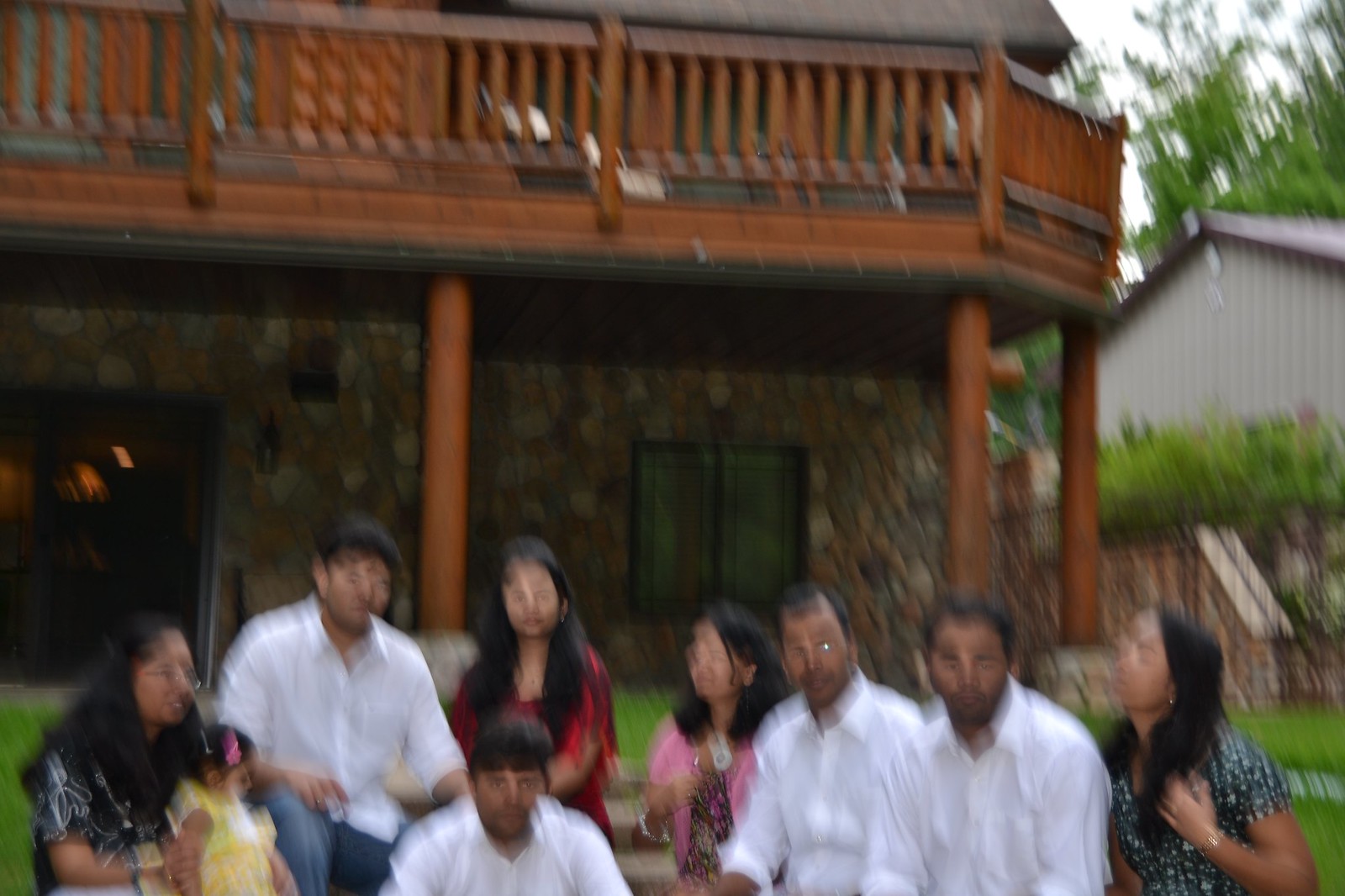A blurry photograph depicts a family gathered outside their home. The significant motion blur and out-of-focus effect make the image somewhat difficult to view, with faces slightly distorted but still discernible. The family consists of nine members, including one child—a young girl dressed in a bright yellow dress. Among the adults, there are four men dressed in white collared button-up shirts and four women wearing dresses in various colors. On the far right, a woman is seen in a green and white dress, next to her is another woman adorned in a pink-colored shawl paired with a black and pink dress. Standing in the middle, a third woman wears a striking red dress, while on the side, the fourth woman is in a black and white dress. The group stands in front of a multi-colored stone-walled building, characterized by a reddish-brown railing and matching wooden pillars extending to the top floor.